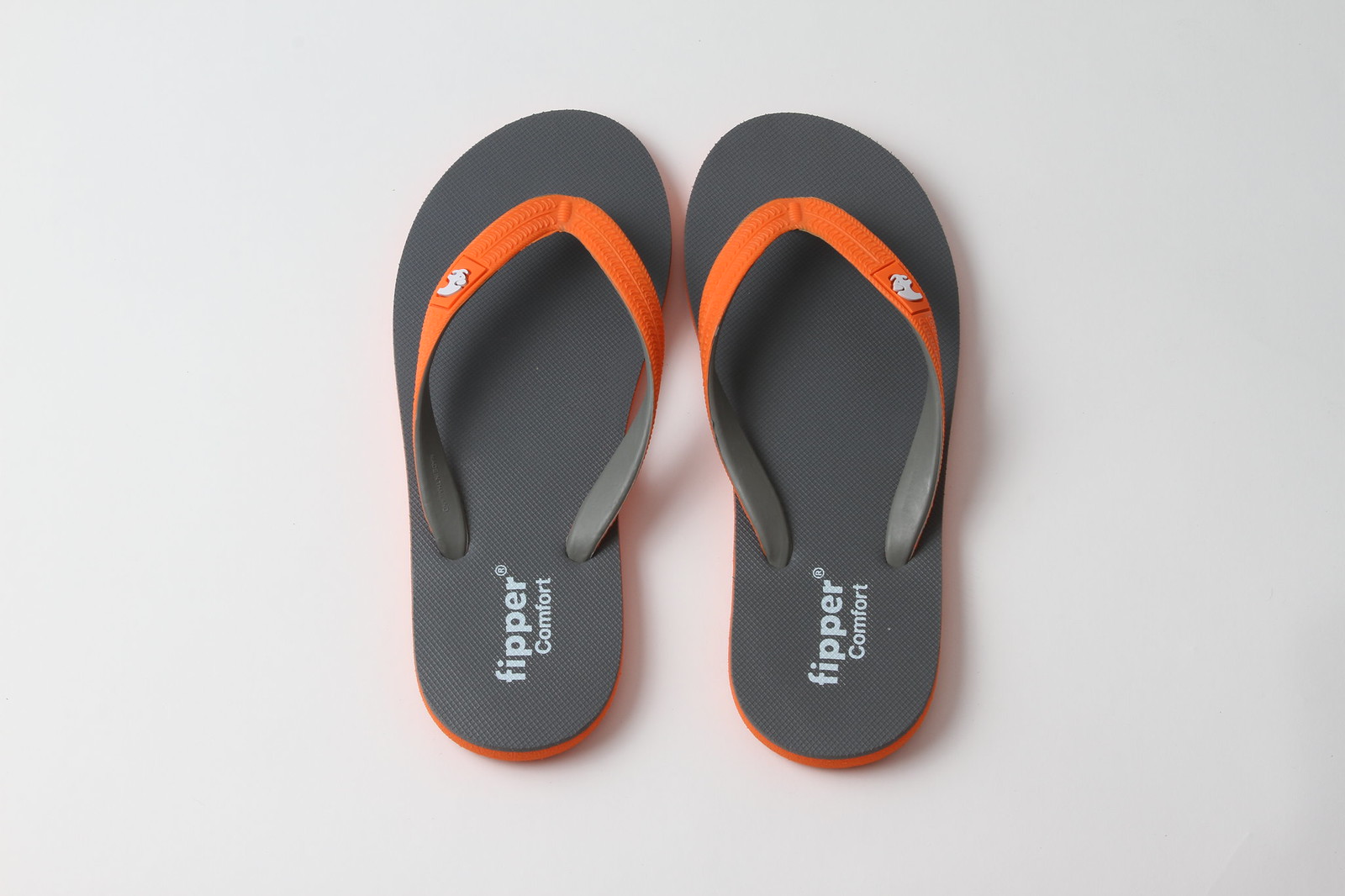The image features a neatly aligned pair of brand new flip-flops centered on a light gray background. Both sandals share a gray sole with "Fipper Comfort" written on the heel. The toe pieces are orange and feature a small white logo, positioned on the left side of the left sandal's strap and the right side of the right sandal's strap. The flip-flops are round at the front and display orange detailing around the outer sole, visible at the back but not the front. The sandals are oriented facing forward, with the background giving a clean, minimalistic appearance to the overall aesthetic.